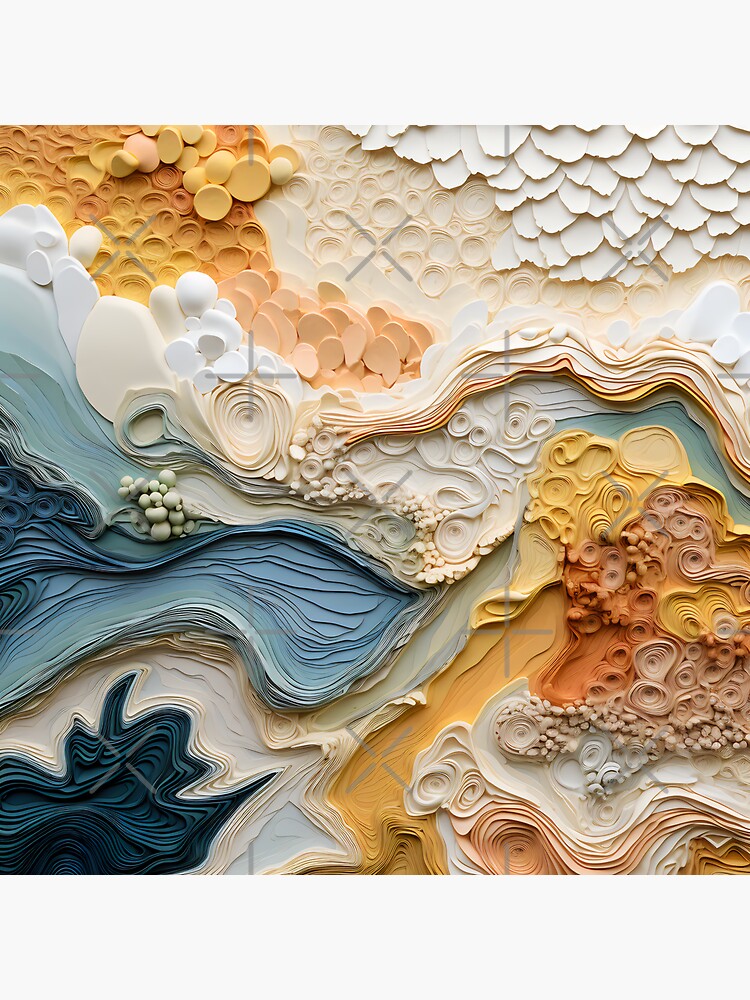This abstract and textured photo showcases a vibrant array of swirling pastel colors and shapes, creating a visually captivating and complex piece of art. On the top left, there's a blend of yellow, orange, and pinkish hues which transitions to a peachy and white area. As your eye moves further down towards the middle left, gradients of blue appear, dotted with circles, lines, and bubbles. The colors and patterns seem to drift and intertwine like currents in a river, with no recognizable pattern, as they create a pastel-like amalgamation of light blues, navies, vanilla, tans, and whites. Some sections appear to have a textured, 3D quality, resembling scales or flower petals, hinting at a possible mixed-media creation underneath a hard surface. The piece is accentuated with sporadic watermarks of pluses and crosses, adding an additional layer of complexity to this unusual and distorted artwork.